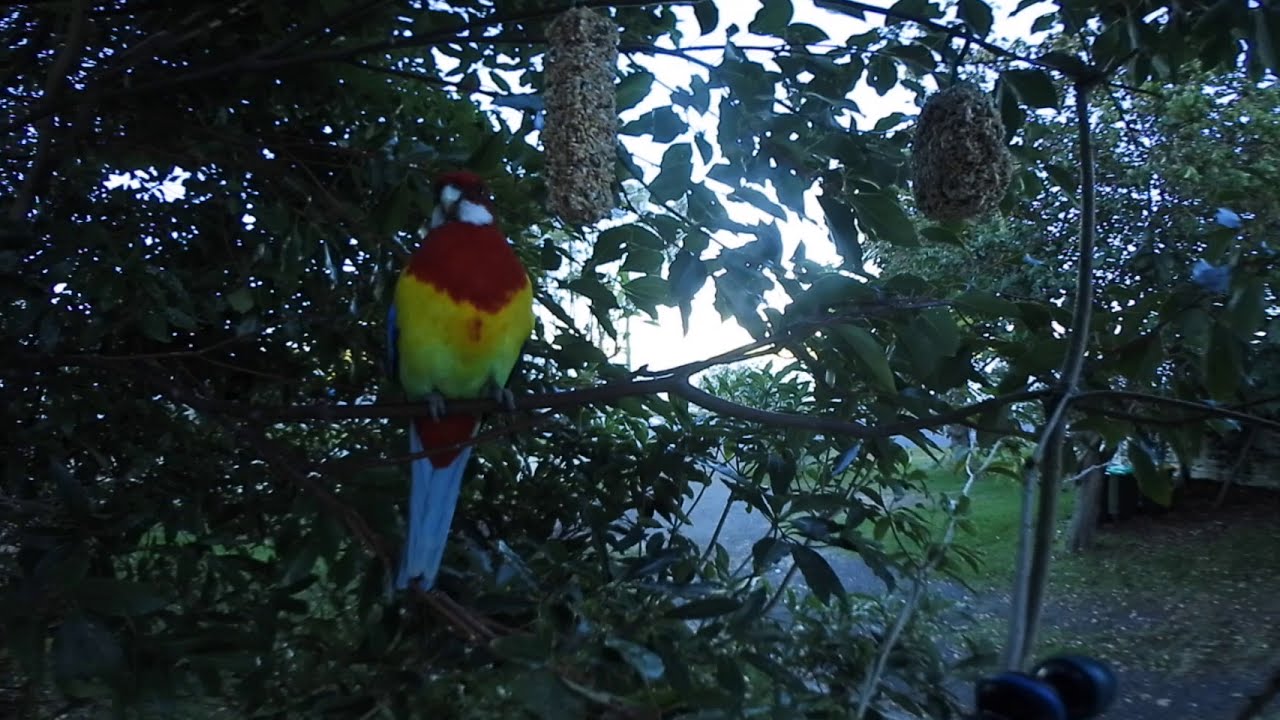In this outdoor photograph taken in a lush, wooded area with abundant green foliage, the main subject is a vibrant bird, likely a tropical parrot. The bird, slightly off-center, is perched on a thin branch amidst a dense canopy of leaves, with sunlight filtering through them. It features a bright red head and collar transitioning to a white area under its beak and a colorful chest that fades from red at the top to yellow and then green. The bird's tail starts with red and white feathers and extends outward, while its blue wings add to its spectacular display. Its feet grip the branch firmly, with additional bird food hanging suspended in front of it. On the far right edge of the photo, partially obscured by leaves, another bird with blue plumage can be seen. The background includes more leafy trees, patches of grass, and a pathway leading out of the wooded area—suggesting a late summer setting under either an overcast sky or one mostly hidden by the thick tree cover.